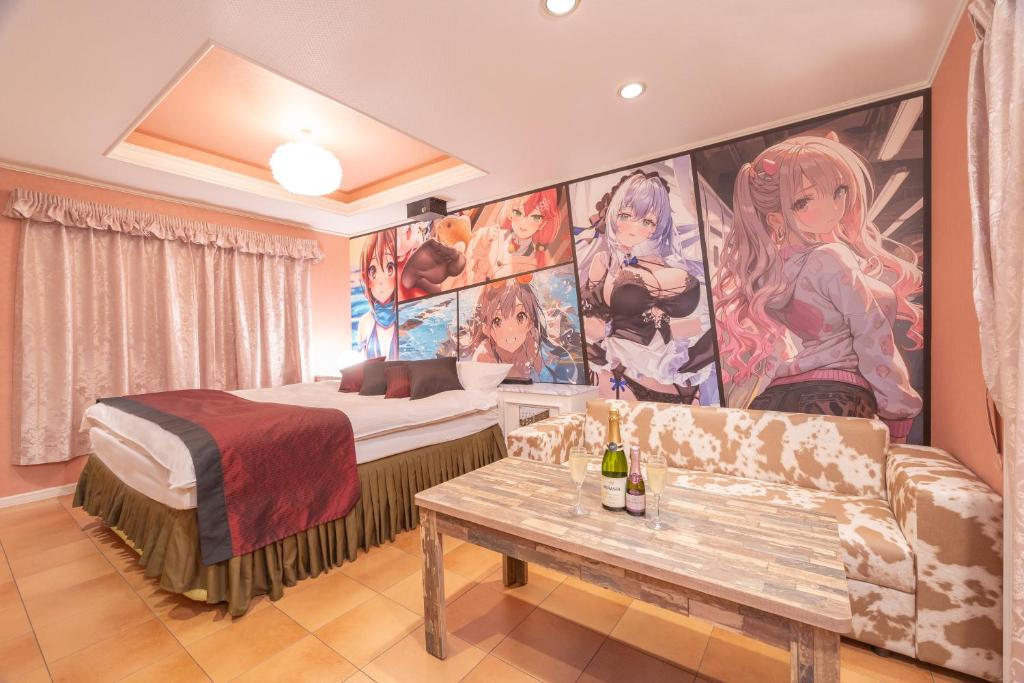This image captures the interior of a bedroom, possibly a hotel room, with a blend of cozy and vibrant elements. The room features a white ceiling and a floor adorned with light brown, almost wooden-colored tiles. Positioned to the left is a queen-sized bed topped with white sheets, an olive green bed skirt, and a red blanket with a black border. The bed also has maroon or wine-colored pillow covers.

Against the back wall, the room's most striking feature is a gallery of anime-style posters. From left to right, there is a redheaded woman facing forward, a pink-haired woman with her foot in a black stocking, an underwater woman, a woman in a sexy maid outfit, and a woman with pink hair wearing a white top, her back to the viewer but with her head turned.

Adjacent to the bed on the other side is a small table holding two wine bottles and two full glasses of wine, situated in front of a brown and white speckled couch. Light pink drapes adorn one side of the bed, and a large ceiling light illuminates the space, adding to the room's bright and lively ambiance.